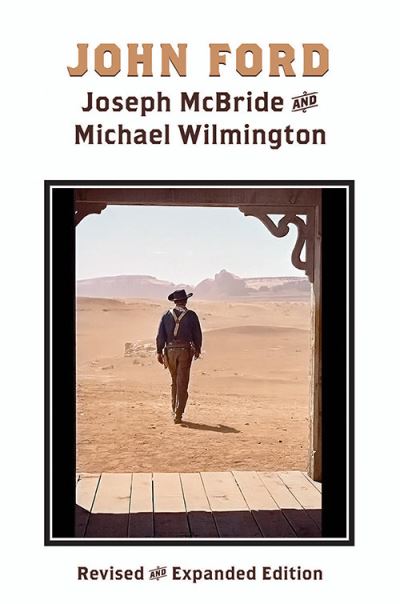The image appears to be a poster featuring a detailed scene in a desert landscape. At the top, large, burnt orange block letters spell out "John Ford," followed by the names "Joseph McBride" and "Michael Wilmington" in dark brown, with their respective initials capitalized. In between these names is a small shadowed symbol indicating "and." Below the text, a vertical rectangular photograph is framed with a black border, followed by a thinner cream-colored border, and an inner dark border. A brown molding with a squiggle design is visible at the top of the frame, suggesting the viewer is inside a building, looking through an open doorway.

The photograph captures a light blue sky and a grayish mountain range extending across the middle. The foreground features a sandy desert terrain extending up to a wooden deck with vertical wood slats. On this deck stands a man with his back to the camera, casting a shadow. He wears a cowboy hat, a dark long-sleeved shirt, tan suspenders, and dark brown pants, resembling a figure from the Wild West. There might also be a belt with an accessory such as a gun on his left side. At the bottom of the image, the text "revised and expanded edition" is displayed, indicating that this is an updated version of a previous work.